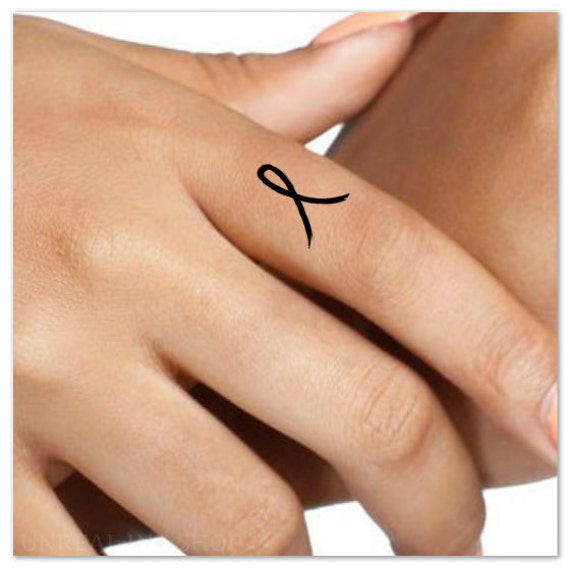This image is an extreme close-up of a woman's right hand with a light tan complexion. The hand is grasping another body part, possibly another arm, although this is highly obscured and cut off in the photograph. The close-up reveals meticulously styled fingernails, with the visible thumbnail painted in an ivory or off-white color. Notably, there is a black ribbon symbol on the back of her index finger, positioned between the lower knuckle and the fingertip. This ribbon appears digitally superimposed rather than being a tattoo, as it contrasts sharply with the natural texture of the skin. The background is a plain white with no distinguishing features, further directing attention to the hand and the ribbon. The image highlights the clarity and smoothness of her skin, devoid of any hairs or distinguishing marks.